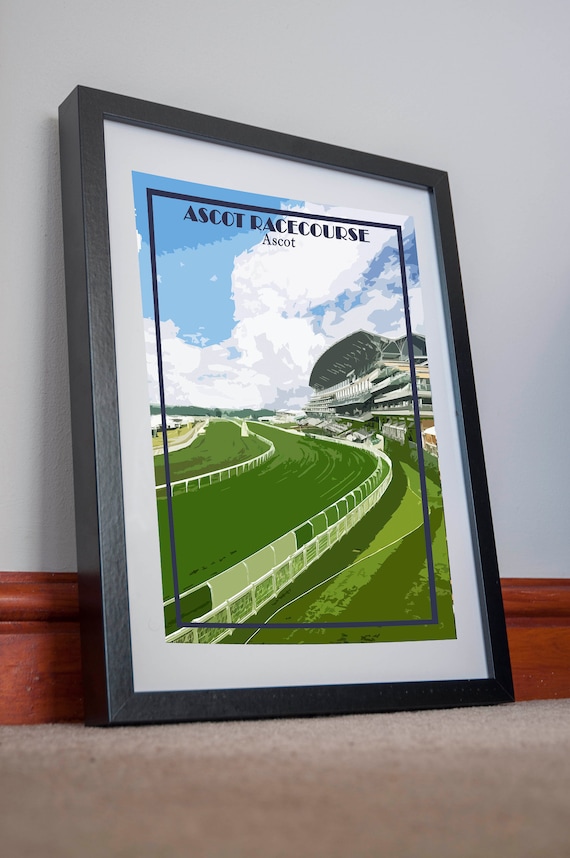The picture is of a framed painting leaning against a blue wall with dark brown wooden trim at the bottom. The painting itself is enclosed in a black frame with a white mat and features a navy blue inner border, creating a layered look. The floor beneath is a light gray color. The artwork depicts a vibrant racetrack scene with lush green grass and a white fence running along the course. Above the racetrack, blue skies with white clouds are visible. A prominent gray and white stadium, approximately three or four stories tall, stands in the background to the right. The top of the painting features large blue lettering that reads "Ascot Racecourse," with a smaller "Ascot" written underneath. On the left of the track, there is a caution area with additional green grass and white railing. The scene is detailed and captures the essence of the racecourse vividly.